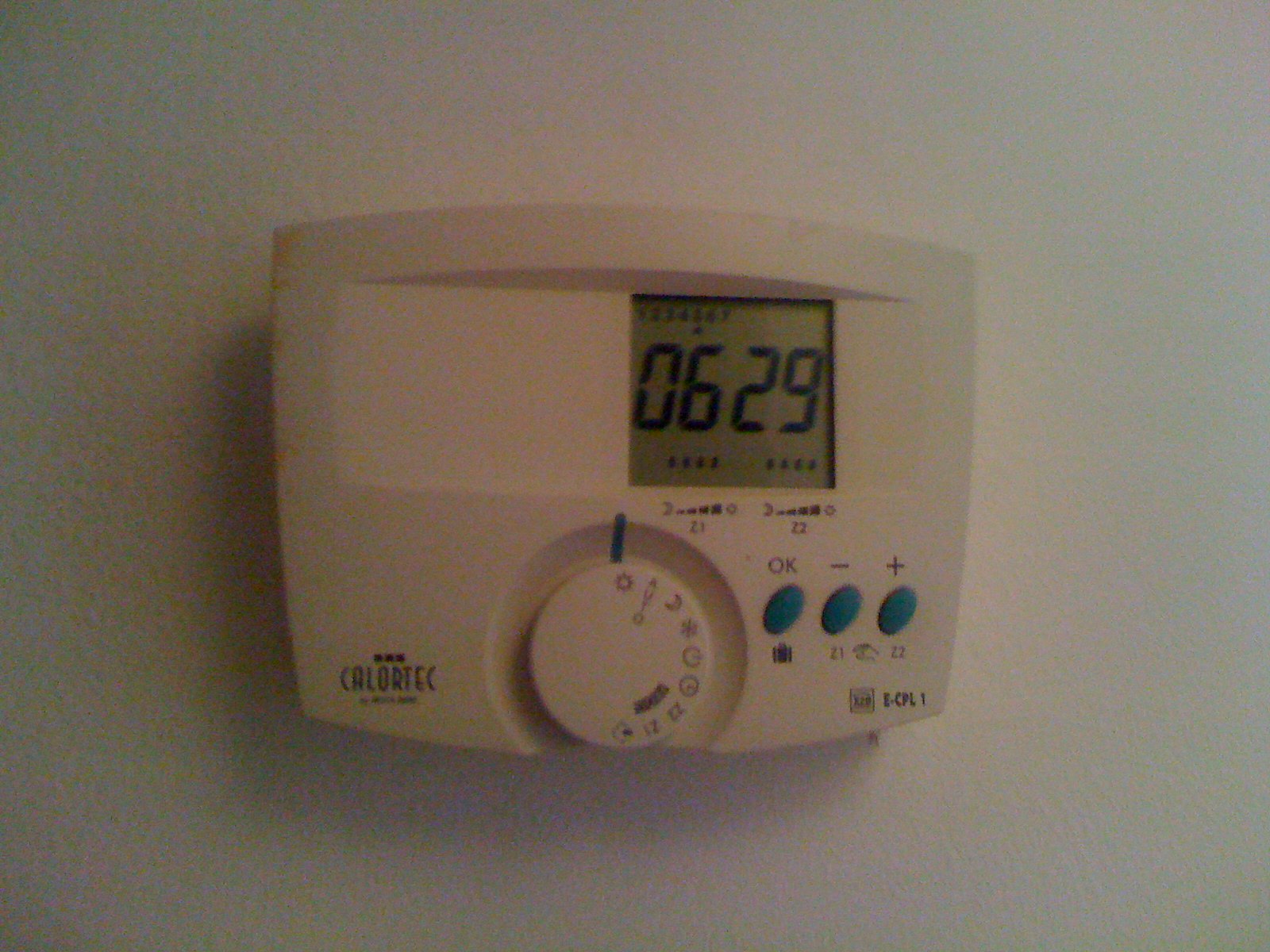A sleek, rectangular white plastic device with elegantly curved edges is mounted on the wall. This object, which closely resembles a thermostat, has the brand name "Calortic" subtly embossed in gray on the bottom left corner. Adjacent to the brand name is a prominent white dial adorned with various symbols, starting with a sun icon, followed by letters, a crescent moon, and other icons encircling its circumference.

To the right of the dial, three small, oval-shaped blue buttons are arranged diagonally. Each button has a clear function: the top button is labeled "OK," the middle button is marked with a minus sign indicating "negative," and the bottom button features a plus sign for "positive."

Dominating the upper half of the device is a digital display, slightly offset to the right, where the numbers "0629" are prominently shown in black.